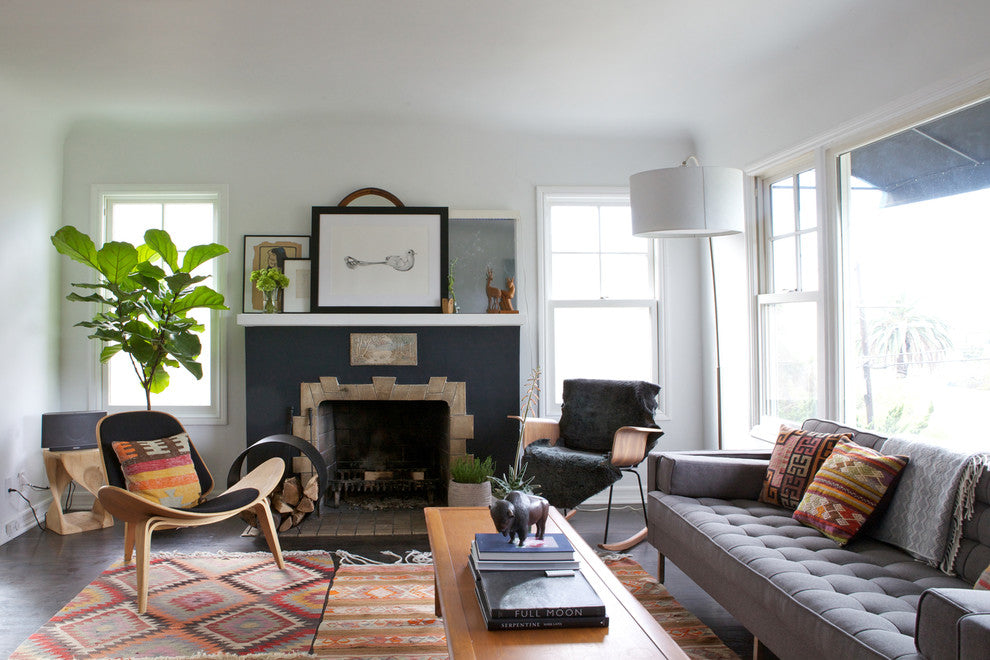This photograph captures a stylishly designed living room with high, white ceilings and light grey walls. The focal point is a centrally placed fireplace crowned with an art piece and flanked by two glass windows. The hearth itself features two small statues and a navy-painted top. There is a large green houseplant beside the left window, adding a touch of nature to the scene.

The room's floor is covered with dark hardwood and two lightly colored, patterned rugs. The rug on the left has a faded Native American-inspired design featuring black outlines and a mix of white, red, orange, and light blue squares. The right rug showcases light brown and orange stripes and supports a light brown coffee table. This table holds a few books and a small bull statue, adding to the rustic yet sophisticated ambiance.

In front of the large window on the right side of the room is a grey sofa adorned with vibrant, multi-colored cushions for a pop of color. To its left is a cream-colored chair also decorated with a similarly colorful cushion. A wooden chair with a grey throw completes the seating arrangement between the sofa and the cream chair. The room bathes in natural light from the large windows, making it bright and inviting. A white lamp in the right-hand corner ensures ample lighting during the evenings. Overall, the space is a harmonious blend of comfort, warmth, and tasteful décor.